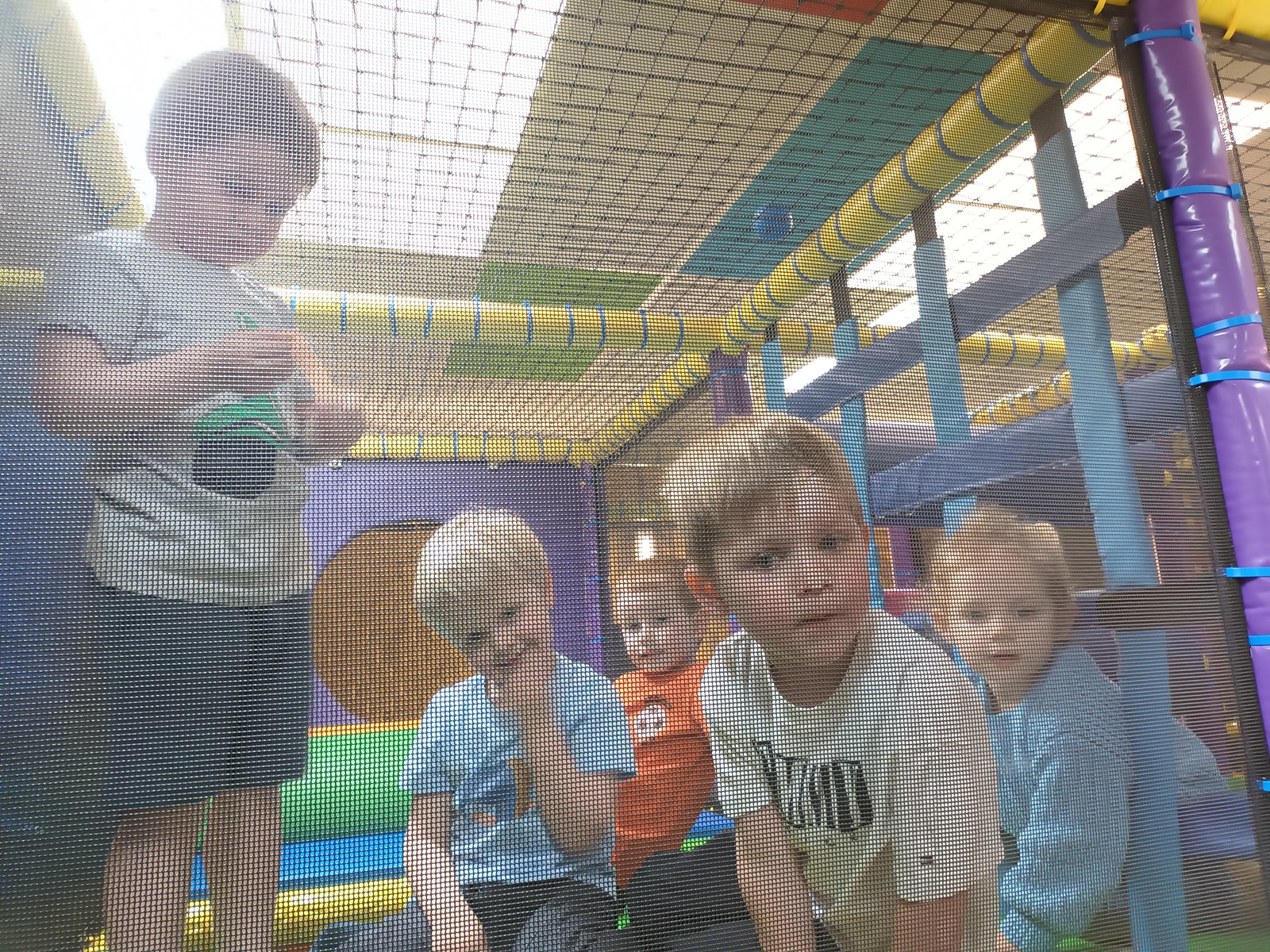This image captures five children playing in an enclosed play area, possibly a ball pit or bounce house, enclosed with black netting and padded rails. The ceiling features a mix of off-white, light blue, and light green rectangular panels with some white lights. The play area includes vibrant and multi-colored tubes, displaying vivid hues like yellow with red lines and a prominent purple tube with blue, metallic straps.

In the front, a blonde-haired child wearing a white t-shirt stands out, while another blonde-haired child behind him is dressed in a bluish sweater. At the far back, a child wearing an orange shirt can be seen. To the left, one child is in a light blue t-shirt, and on the far left, another child sports a beige t-shirt with gray shorts. All the children appear to be looking at the camera and seem very happy. The image is slightly blurry and hazy, capturing a lively and joyful moment amidst a colorful and dynamic play environment.